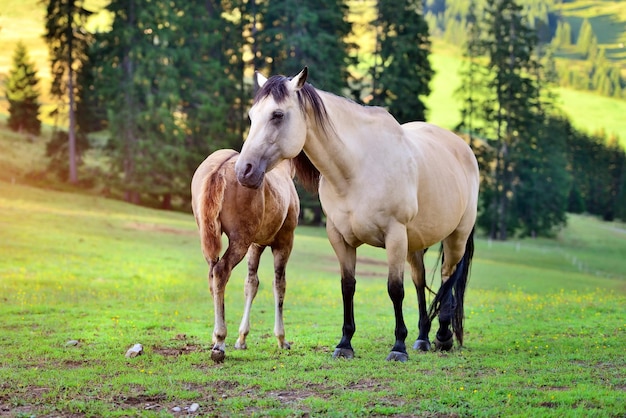In this vibrant outdoor photograph taken on a sunny day, we see a serene scene set on lush, green, rolling hills dotted with evergreen trees. The natural sunlight, either at sunrise or sunset, baths the hills in a warm, golden glow, particularly in the background. The image features two horses—a muscular, tan-colored mare with striking black points on her legs, tail, mane, ears, and facial features, and her light brown foal with white lower legs. The mare, standing at an angle but facing the camera, exhibits a strong and defined chest, while her foal walks away from the camera, showing only its rear end and tail. Scattered along the pathway and on the hills are bits of litter, adding a touch of realism to the idyllic scene. The sunlight’s angle casts a beautiful highlight and shadows, enriching the image's depth and detail.